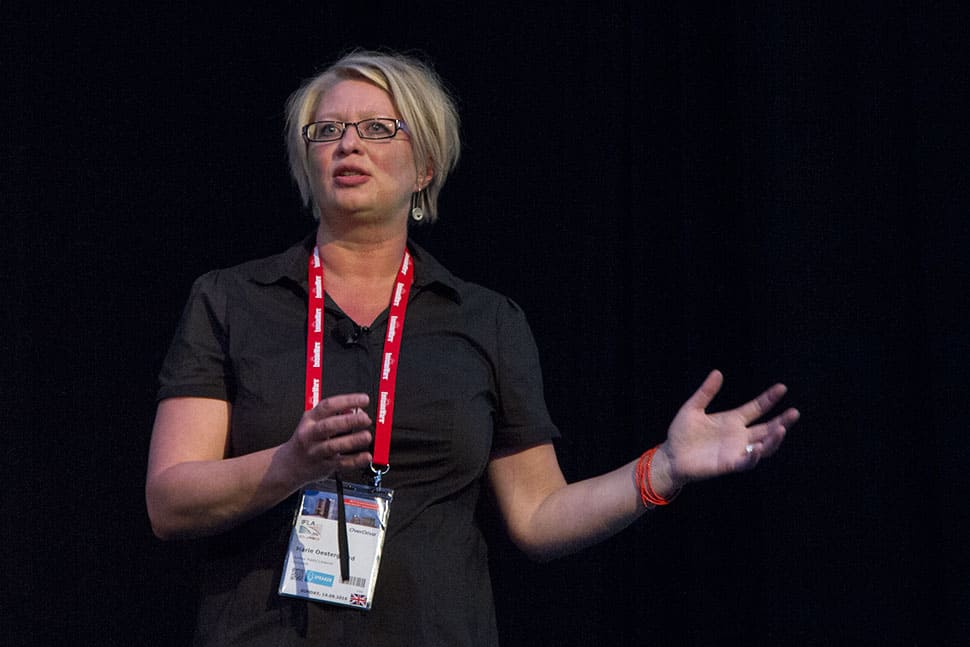In the photo, a middle-aged Caucasian woman is captured in the middle of delivering a speech or presentation against a completely black background. She has short blonde hair styled in a pixie cut or short bob and wears black rimmed glasses. Her attire includes a professional-looking black short-sleeve blouse, which almost blends into the dark backdrop. Around her neck, she has a red lanyard displaying an identification badge in a clear plastic holder, possibly indicating her name and featuring the UK flag, hinting at a press conference or formal event. On her left wrist, she wears a silver ring and multiple orange or red bracelets, adding a subtle touch of color to her subdued outfit. She is gesturing with both hands open towards the right side of the image, while looking up towards the left, seemingly engaging with her audience. The lighting highlights her, making her the clear focal point of the image.